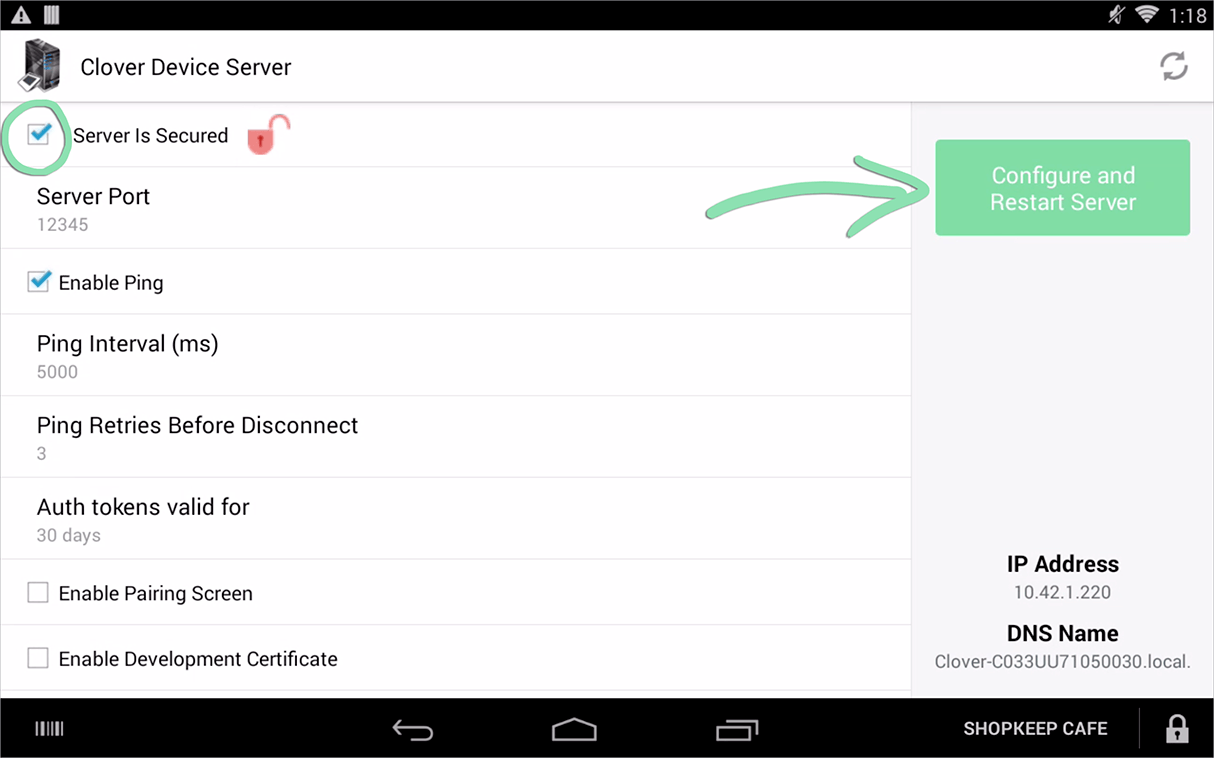The image is a screenshot of a landscape-oriented website or tablet interface. At the top, there is a thin status bar displaying a gray warning icon—a triangle with an exclamation point inside—indicating an alert or notification. Adjacent to this are four vertical parallel lines, likely representing the signal strength, and icons showing that the sound is muted and full Wi-Fi connectivity. The time displayed is 1:11.

The main content area features a heading that reads "Clover Device Server," accompanied by an icon resembling a computer tower. Below this, a green-outlined square with a blue check mark indicates that the server is secured. Adjacent to it is a red lock icon with an open padlock, accompanied by the text "Server Port: 12345."

Further down, another blue check mark inside a square indicates that the "Enable Ping" option is activated. There are additional configurations detailed as follows:
- Ping intervals (in milliseconds)
- Ping retries before disconnect (set to 3)
- Authorization tokens valid for 30 days
- Options to enable pairing screen, document, and development certificate

At the bottom, navigational icons include a back arrow, home button, tab switcher, ShopKeep, Cafe, and a lock icon, all in black with white text.

To the right, a spring green arrow points to a rectangular button, also in spring green, labeled "Configure and Restart Server," suggesting the primary action available for the user.